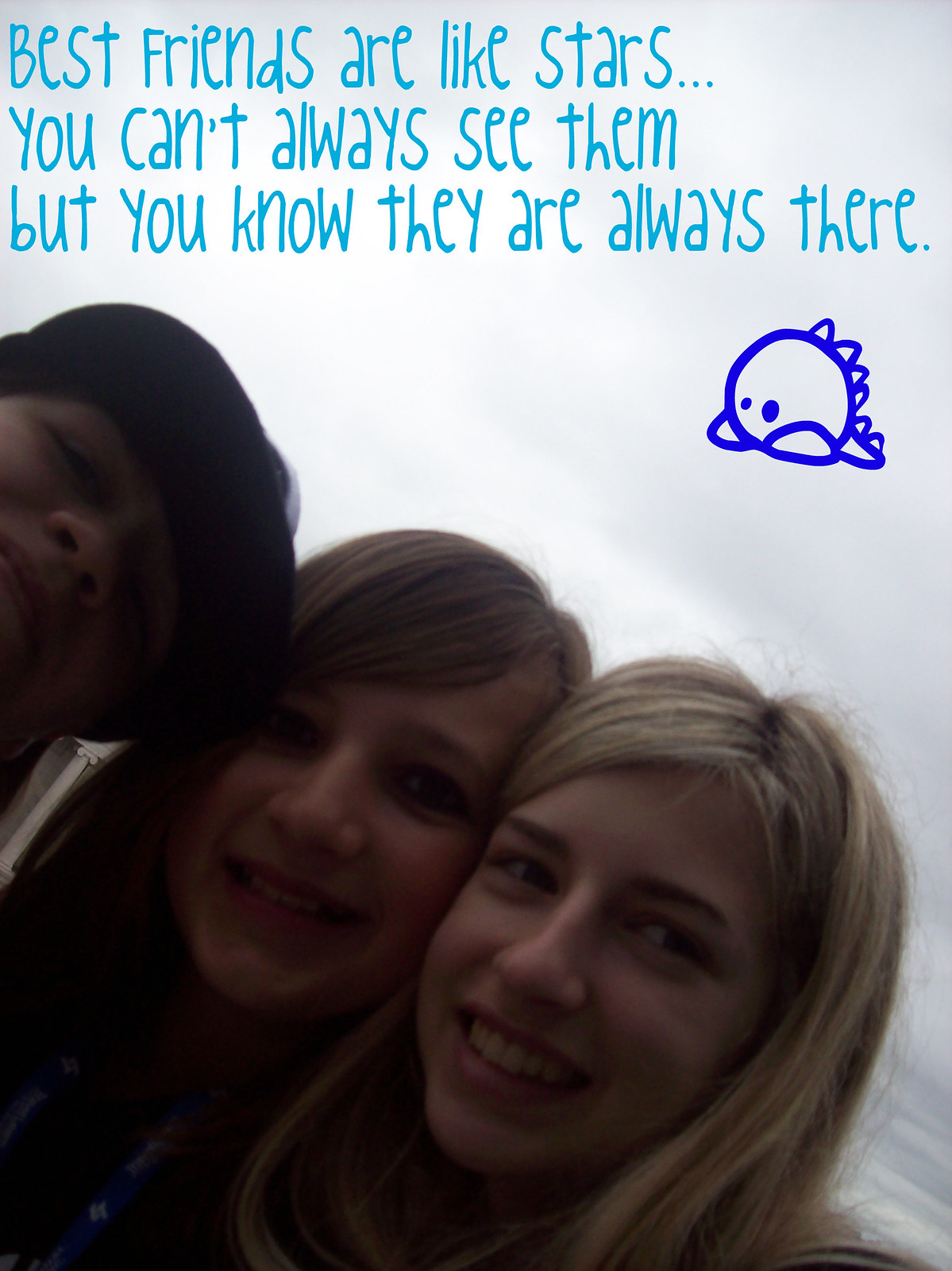This image features three smiling teenage girls who appear to be around 13 or 14 years old. The girl on the right has blonde hair, the girl in the middle has long brown hair, and the girl on the left is wearing a baseball cap, with her face and hair partially out of the frame. They are indoors against a white background that seems to be a paper or sheet, but the dim lighting obscures much detail. At the top of the image, in light blue text designed to look like a girl's handwriting, is the caption: "Best friends are like stars. You can't always see them, but you know they are always there." Below the caption, there's a cute, hand-drawn illustration of a blue dinosaur.